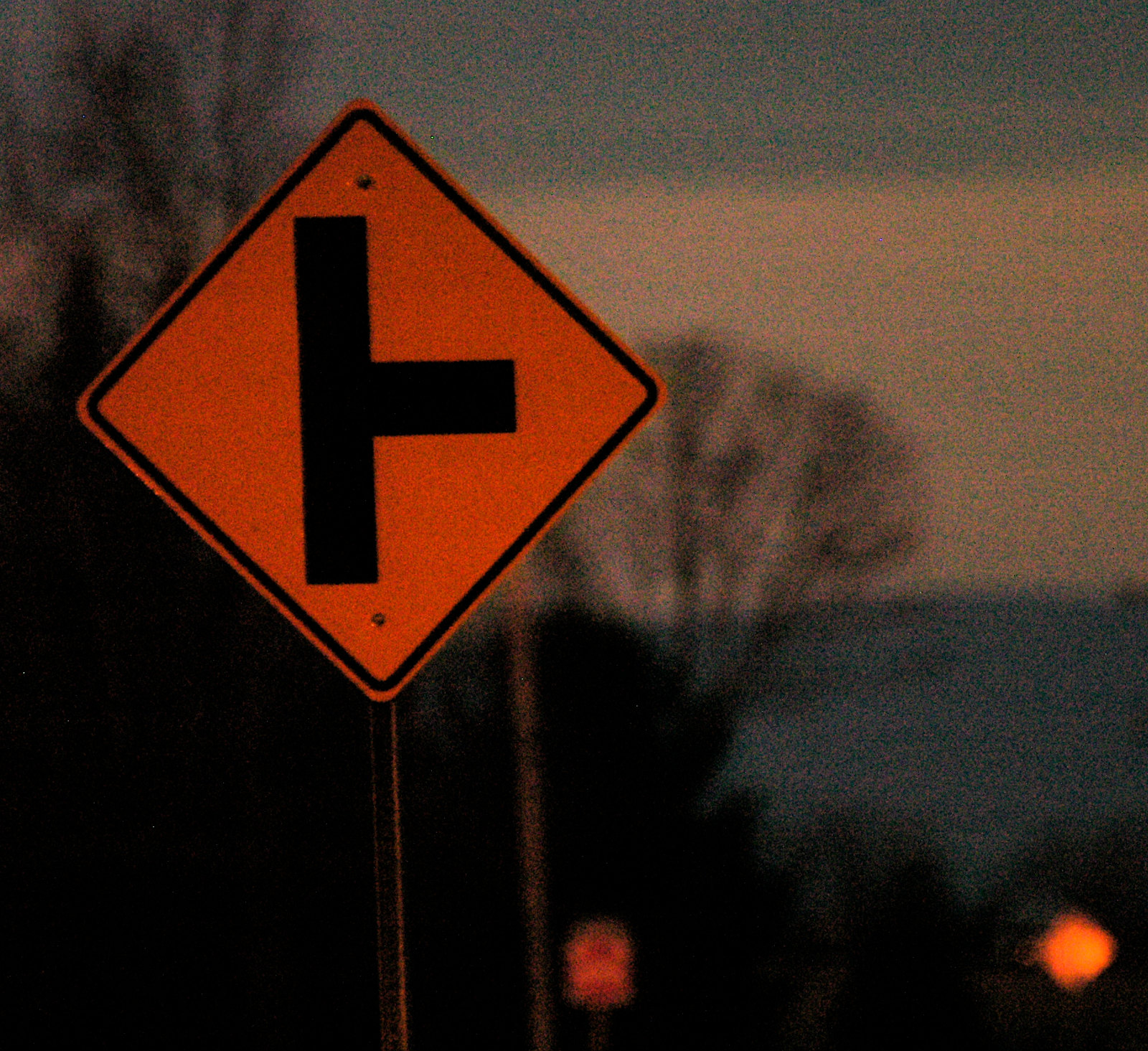The photograph, taken during dusk or early nighttime, prominently features a diamond-shaped road sign on a metal post, located on the side of a road. The sign, which is typically yellow, appears orange in this image. It depicts a straight vertical line with an adjoining line to the right, forming a T-shape on its side, indicating an upcoming intersection. In the distance, a blurry stop sign is faintly visible. The sky shows a gradient of blue with scattered white clouds, and tree branches are also present, contributing to a grainy texture that adds a unique atmospheric quality to the image.